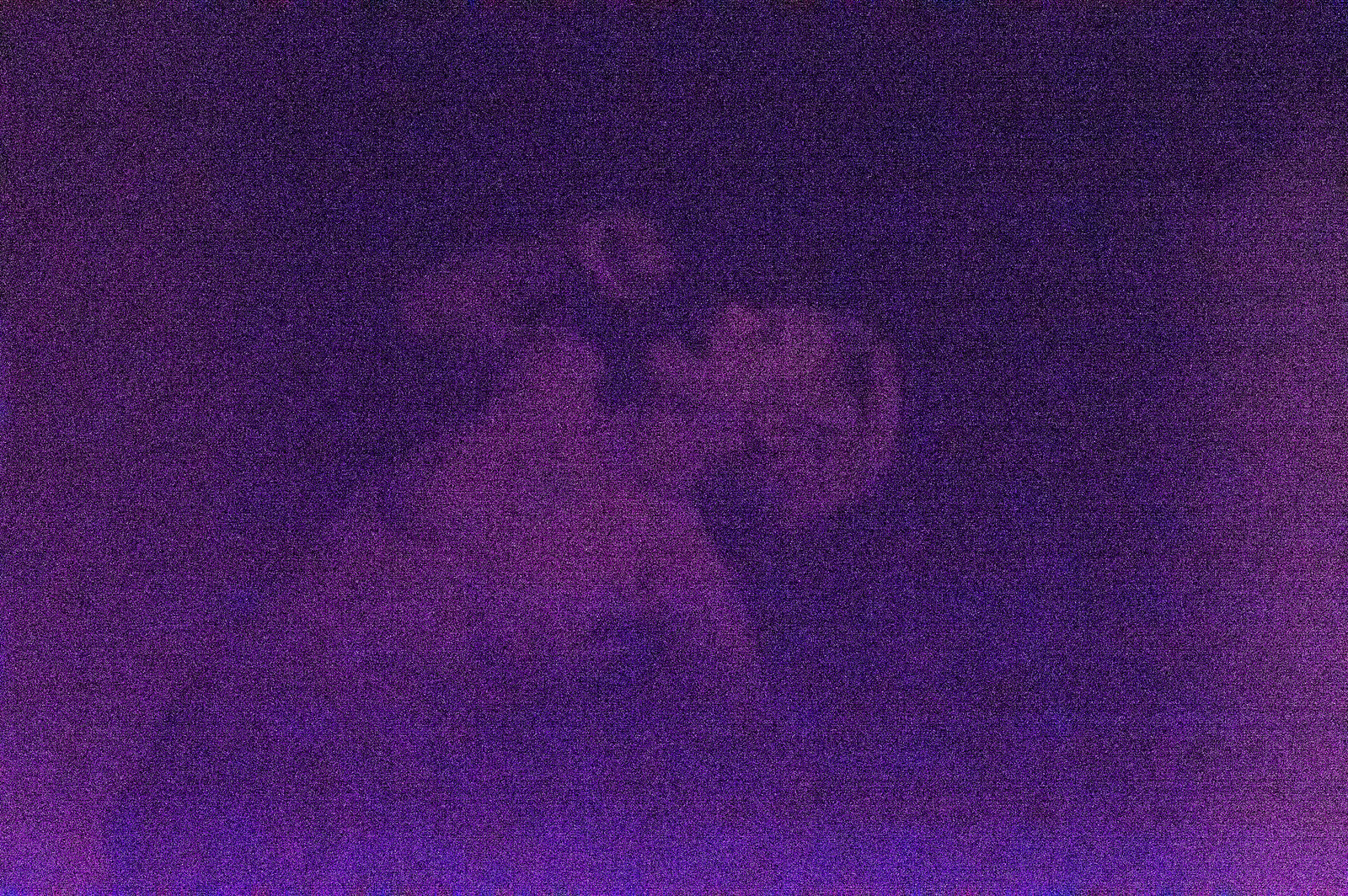The image depicts a high-resolution, staticky purple scene with varying hues from dark to light. At the center, a detailed silhouette of a person with short hair is visible, appearing to scream or shout with their mouth wide open. The figure, seemingly not wearing a shirt, reveals partially visible breasts and nipples. The person is slightly bent over to the right, as if stretching or turning their body, with their left arm raised and bent towards their mouth, possibly mimicking the act of drinking. The background and the figure blend in various shades of purple, contributing to the overall eerie and dynamic atmosphere of the image. The staticky texture adds to the sense of movement and emotional intensity.